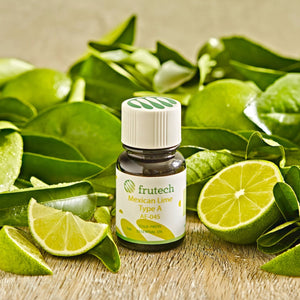The photograph features a dark glass bottle with a white cap, prominently labeled with "Freetech" in green letters, and underneath, "Mexican Lime Type A" in lime green. The label also includes the code "A F 0 4 5". Surrounding the bottle are numerous vividly colored lime slices, some halved and others quartered, along with waxy green lime leaves elegantly scattered about on a wooden brown surface. The background showcases an arrangement of green hues, featuring dark greens, lime greens, and yellow greens, giving the scene a fresh, vibrant feel. The setting is completed by the texture of the wooden surface and a cream-colored wall in the background.